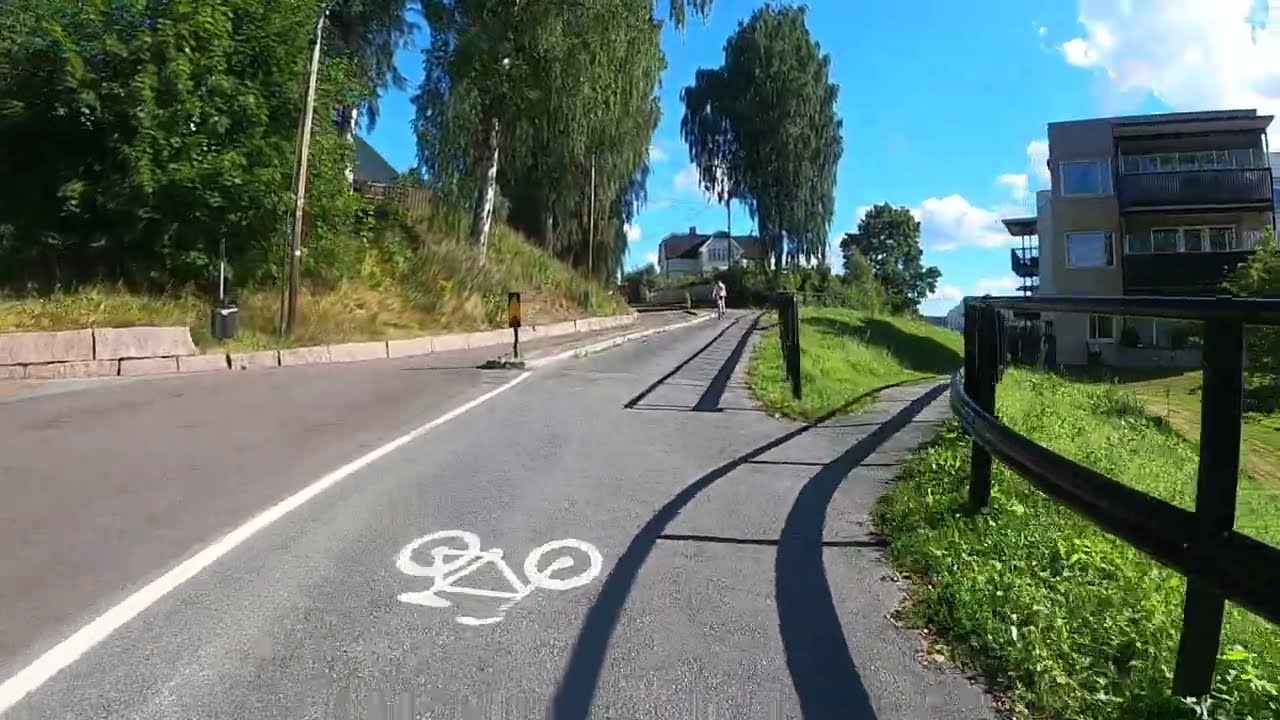This photograph captures a road prominently featuring a green bike path marked by a white painted bicycle symbol, designating it exclusively for cyclists. The path diverges further ahead, splitting into two, with one branch curving to the right. On the road, a cyclist dressed in white can be seen riding towards the viewer. To the right side of the road, there's a black metal railing and several buildings that appear to be houses or possibly apartment buildings. This side is also bordered by grass and scattered trees. Surrounding the green bike path, the left side of the road is embraced by a wooded area with a variety of trees, including evergreens, and there’s a glimpse of a modern house, possibly a mansion, nestled among the foliage. The sky is a vivid blue adorned with scattered white clouds, suggesting a bright and beautiful day.